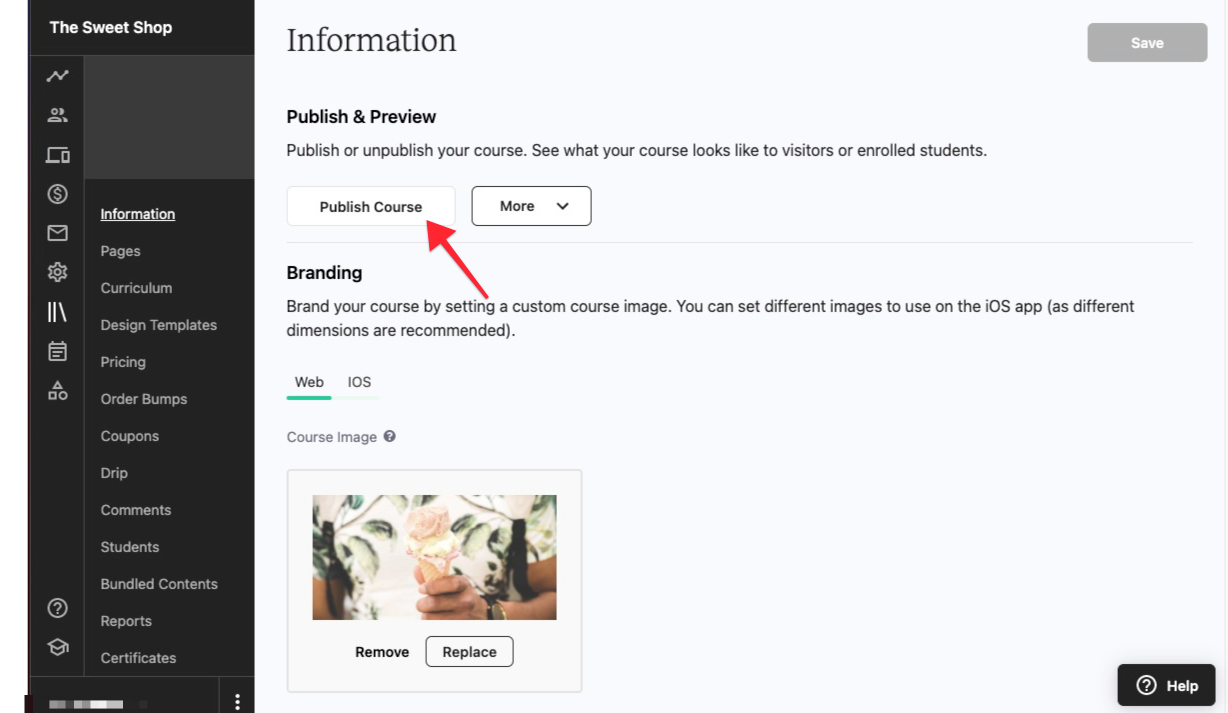Here's a refined and detailed caption based on the provided description:

---

**Dashboard Interface of "The Sweetshop" Online Course Management System**

This black-and-white interface belongs to "The Sweetshop." On the upper left corner, the title "The Sweetshop" is prominently displayed. Adjacent to it is a comprehensive left navigation bar divided into various sections with gray placeholders and labeled text such as Information, Pages, Curriculum, Design Template, Pricing, Order Bumps, Coupons, Drip, Comments, Students, Bundled Contents, Reports, Certificates, and more. Further left is a vertical strip featuring icons representing different functions: a zigzag pattern of dots and lines, two users, a computer, a cell phone, a money sign, an envelope, a settings cog, three lines leaning on each other, a calendar, a triangle over a square and a circle, a question mark, and a graduation cap.

The main workspace displays sections titled Information, Publish and Preview. Here, users can publish or unpublish their courses or preview how the courses appear to visitors or enrolled students. Below these options, there are buttons for saving (gray button) and publishing the course (with a red-drawn arrow pointing to it for emphasis). Additionally, there's a "More" button with a dropdown menu and a "Branding" section encouraging users to set a custom course image. It also notes the capability of setting different images for use in the ISO app, highlighting the platform's versatility and customization offerings.

---